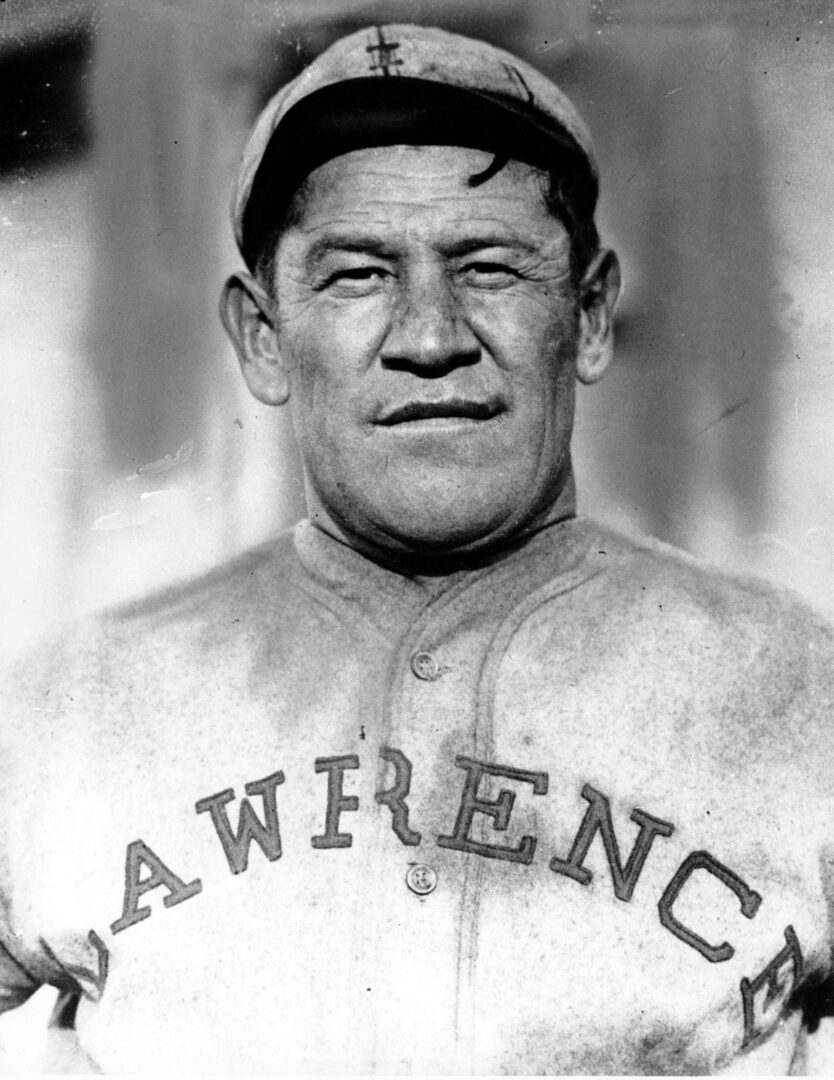This is a vintage black-and-white portrait photograph of the legendary baseball player Jim Thorpe, taken in the early 1900s. The image is oriented in portrait format and captures Thorpe from the top of his head to mid-chest. He is facing the camera with a squint and a slight, half smile, lending a rugged and masculine intensity to his expression. His facial features are distinctive, with a broad, rectangular face, a wide nose, and a square, prominent chin. His dark curly hair peeks out from under a white cap with a short black bill. Fine lines mark his forehead and frame his eyes, adding to the weathered look of his skin.

Thorpe is clad in a light-colored baseball uniform buttoned all the way up to the collar, which appears to be made of wool. The jersey features the name "LAWRENCE" in bold, slightly curved text across the chest. However, due to the positioning of the buttons, there is a gap right down the middle of the 'R,' making it resemble an 'F' at first glance. The background is out of focus, consisting of a blurred mix of gray hues and abstract shapes, with a notable black square in the upper left corner. This enhances the subject's prominence and adds to the photograph's vintage aesthetic.